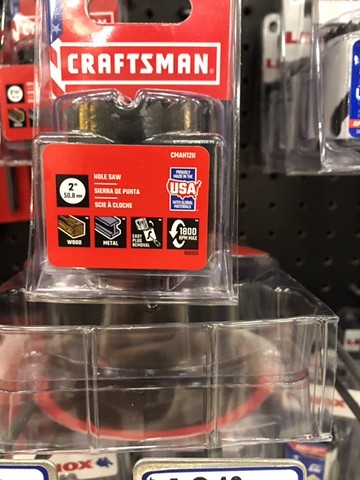This image showcases a package of multi-tool blades manufactured by Craftsman. The blades are encased in a clear plastic packaging with a prominent blue label. The label prominently displays the Craftsman brand name and provides detailed information about the blade's cutting capabilities, including small icons that indicate it can cut wood and metal. The label also mentions an operational speed of 1800 revolutions per minute (RPM). The Craftsman packaging is placed atop another type of plastic packaging with an orange ring visible, though its contents are unclear due to blurring. Additional packaging and cutting equipment, possibly also from Craftsman, are visible in the upper-right corner of the image. The overall scene suggests a variety of cutting tools and accessories intended for multipurpose use.